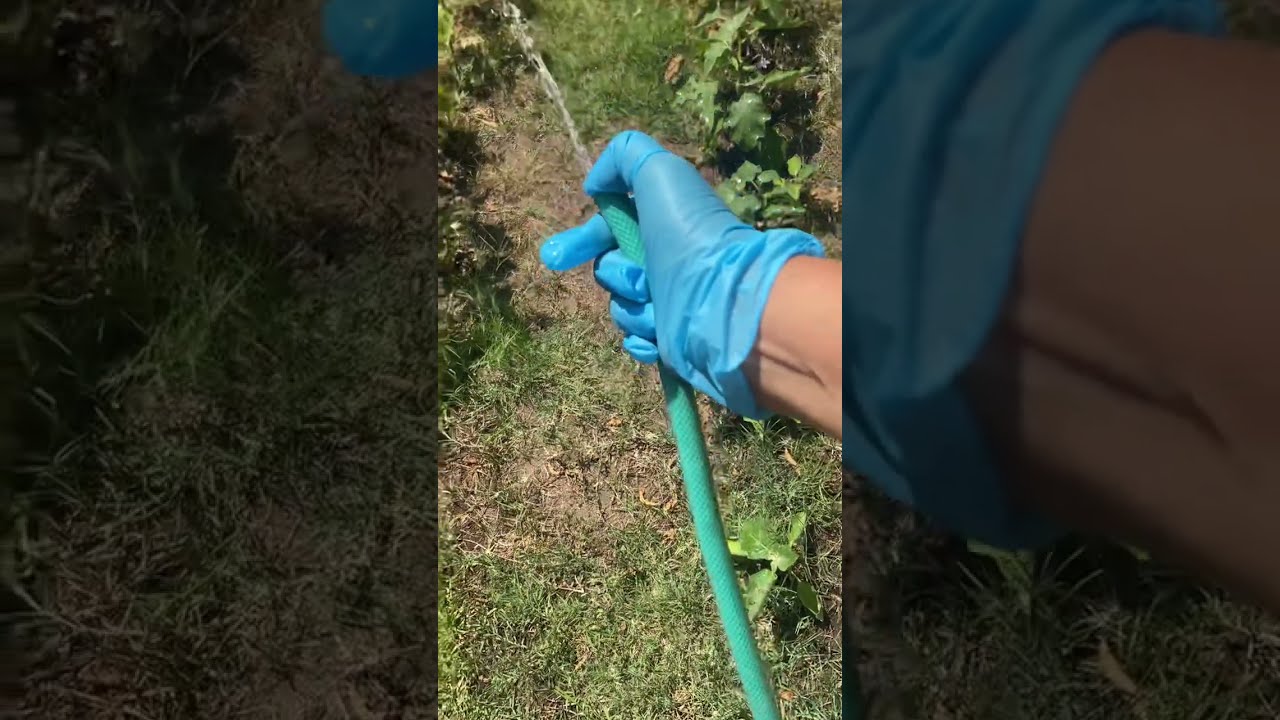The vertical cell phone image depicts a Caucasian man's right hand, covered with an oversized blue latex glove, holding a thin, light green garden hose. The hose lacks a nozzle, so the man uses his thumb to control a thin stream of water spraying onto a sunlit, grassy area below. The grass, appearing predominantly tan and yellow with patches of gray and some isolated green areas at the edges, looks dried out and parched. Surrounding the central image, the background consists of the same picture zoomed in and faded, showcasing close-up views of the dry grass on the left and a portion of the blue-gloved wrist on the right. On the right side, there are visible potted plants with dark soil, while another potted plant might be hinted at on the left. Weeds sporadically emerge from the ground, indicating a somewhat neglected lawn.